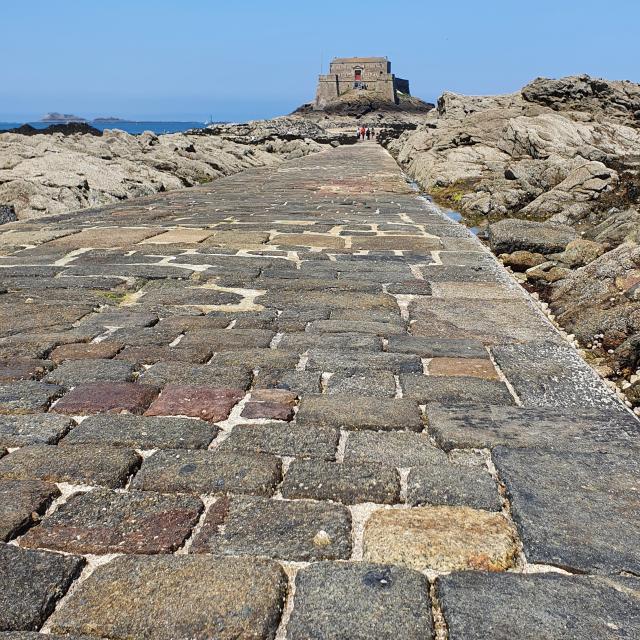This well-lit outdoor photo captures a detailed view of an ancient, cobblestone pathway leading up to a large, fortress-like structure. The pathway is composed of irregular, hand-carved stones in shades of gray, red, and tan, bound together with light-colored grout. On either side of the pathway, jagged, gray rocky cliffs and moss-covered stones rise steeply, creating a dramatic corridor. The imposing stone building at the end of the path, reminiscent of a castle, stands square-shaped with large pillared walls and appears to be a popular tourist spot. A distinctive red door marks the entrance to this ancient structure, which towers about four to five stories high. In the far distance, a beautiful sea with a ship sailing on it and clear blue skies can be seen, adding to the picturesque setting. Near the end of the path, at least four people are visible, with one notably wearing a red shirt. The scene is enhanced by subtle details such as water condensation along the edges of the pathway, indicating the aged and weathered nature of this historic site.